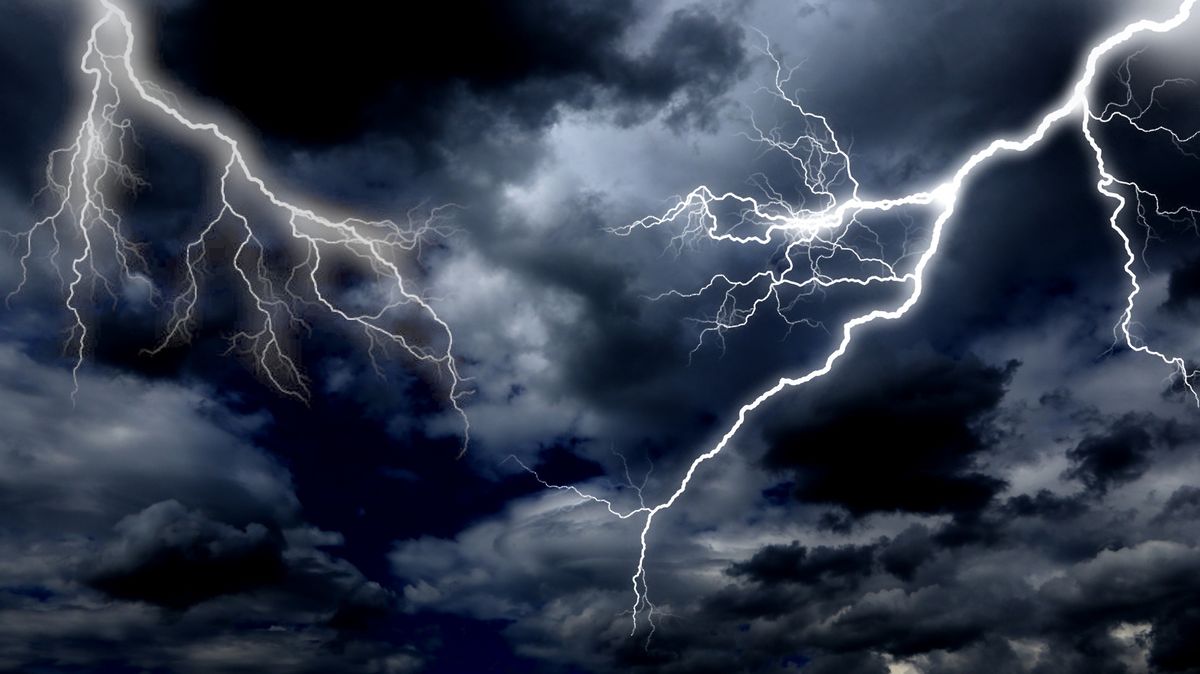This captivating image, which could be either a photograph or a meticulously crafted digital render, captures a dramatic nighttime thunderstorm with powerful lightning strikes. The night sky features a stunning contrast of deep blue and black with dense storm clouds, exhibiting a mixture of textures — from ominously dark to patches of lighter gray. Prominently, two intense streaks of lightning dominate the scene, starting from the upper corners of the image. One yellowed lightning bolt descends diagonally from the upper left, while another bright white bolt crackles downward from the upper right, both almost converging in a complex, intertwined display of raw energy. The lightning, with its jagged, branching patterns, spreads across the sky in a spectacularly intricate web, illuminating the clouds and showcasing the storm's fierce intensity. The photograph is angled upwards, enhancing the grandeur and immediacy of the natural phenomenon, making the viewer feel as though they are witnessing the raw power of nature firsthand.